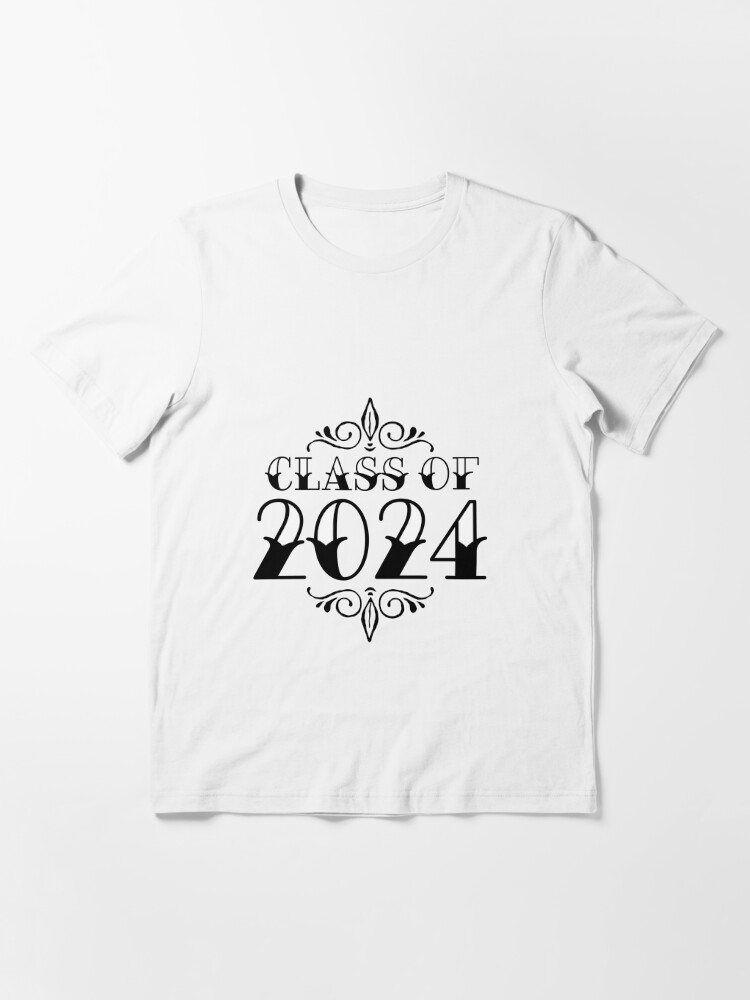The image features a short-sleeved, plain white t-shirt laying flat on a plain white surface, casting a soft drop shadow. The shirt, which has slight wrinkles, is adorned with the text "CLASS OF 2024" in an elegant, fancy font. The text is all in capital letters, with the bottom half solid black and the top half outlined in black and filled with white. Above and below the text are intricate, black and white designs consisting of curly, swirly patterns, along with leafy and diamond-shaped elements, enhancing the celebratory theme of the shirt. The t-shirt has a standard U-shaped neckline, not very deep, and is designed to cover most of the upper body except for the arms due to its short-sleeved nature.